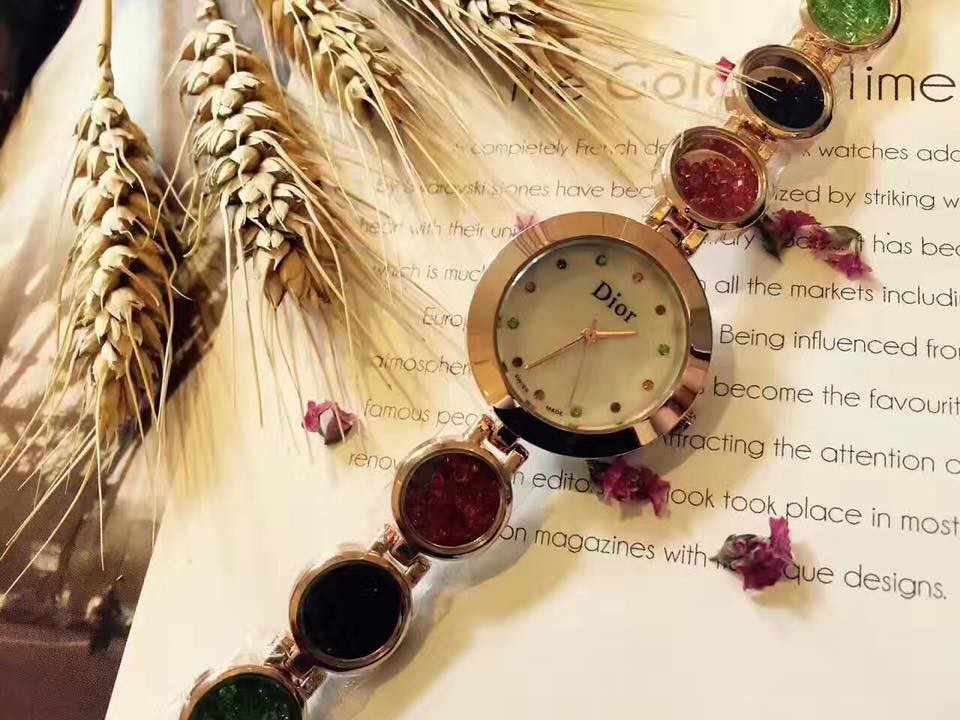This photograph features a luxurious Dior watch displayed atop a piece of paper, with strands of grain-like plants positioned in the upper left corner. The watch, elegantly set to 1:35, boasts a round, gold analog face adorned with various colored crystals in place of numbers. The bracelet consists of gold circles embedded with more gems in vibrant hues of red, purple, and green. The piece of paper beneath the watch contains text discussing the creation and unique design of French watches, although much of the writing is obscured. Violet petals can be seen underneath the watch, adding a delicate touch to the composition. The entire image presents a sophisticated interplay between high fashion and natural elements.